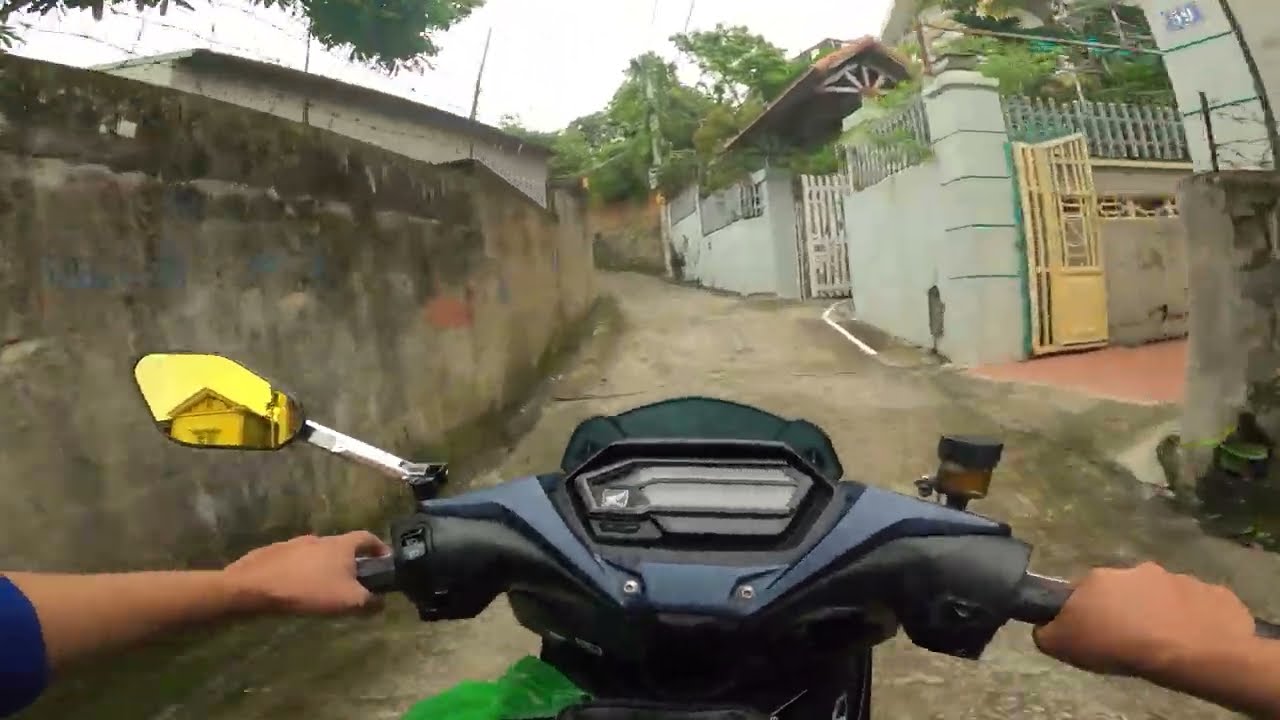The photograph features a moped rider with caramel-colored skin, possibly South Asian, firmly gripping the black and navy blue handlebars of their vehicle. The rider, dressed in a blue-sleeved shirt, navigates a narrow, stone-paved alley. The left side of the moped has a tinted yellow rearview mirror. The street, lined with Asian-style architecture, includes a mix of stone walls and gates leading to grand houses surrounded by lush greenery and trees. The scene, set during an overcast day, captures the aged, somewhat rundown ambiance of the area, hinting at locations like the Philippines or India, with its mud-streaked walls and varied gate colors.